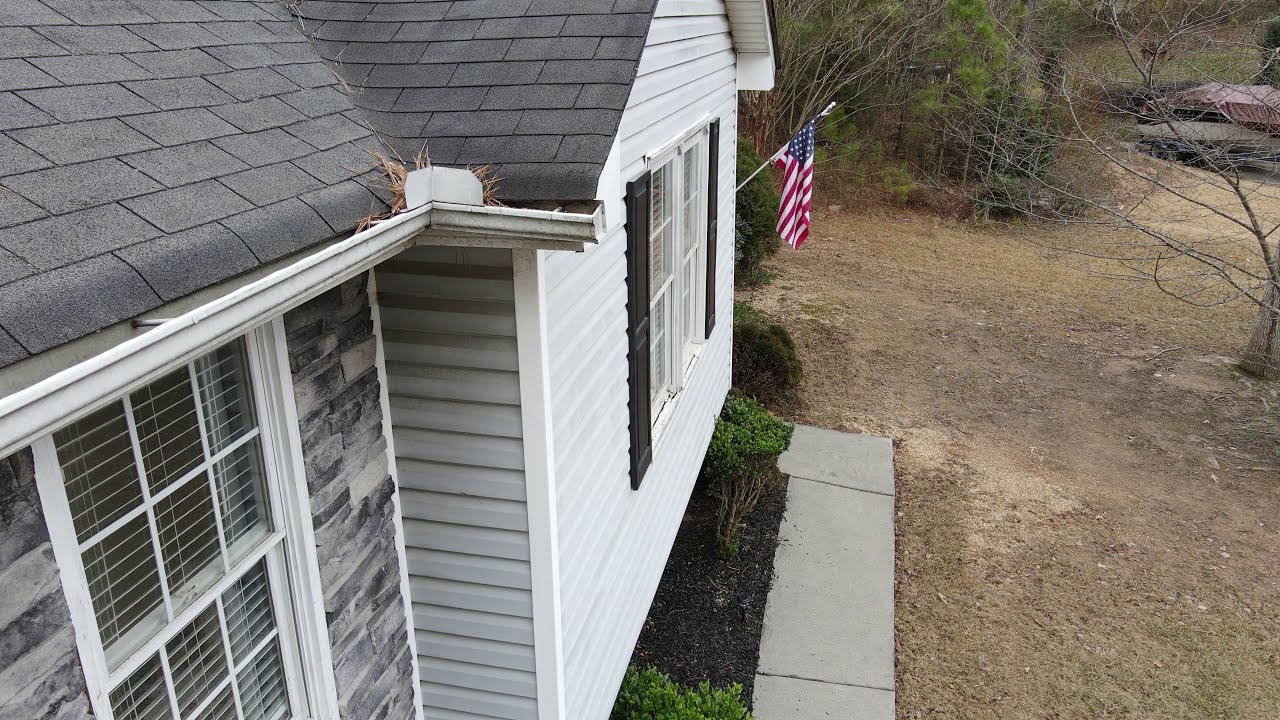This photograph, likely taken from a drone about five feet away and slightly above the midpoint of the roofline, captures a detailed side view of a house set in a rural area. The house features white and gray siding, complemented by black trim around the windows and white blinds within. There's noticeable stonework with a palette of white, gray, and black. The roof is composed of black shake tiles, and a white rain gutter runs along the edge, which is clogged with brown pine needles. 

An American flag is prominently displayed on the corner of the house, adding a touch of patriotism to the scene. Below, there's a short stone walkway that traces the perimeter of the house. In front of one window, two small plants have recently begun to sprout. The yard is characterized by an uncared-for, brown dirt surface, and sparse, small green bushes, set against a backdrop of trees and scattered leaves. To the right of the house, the landscape extends into a natural, tree-filled area, suggesting a stream might be nestled in the background, further adding to the rural charm of the setting.